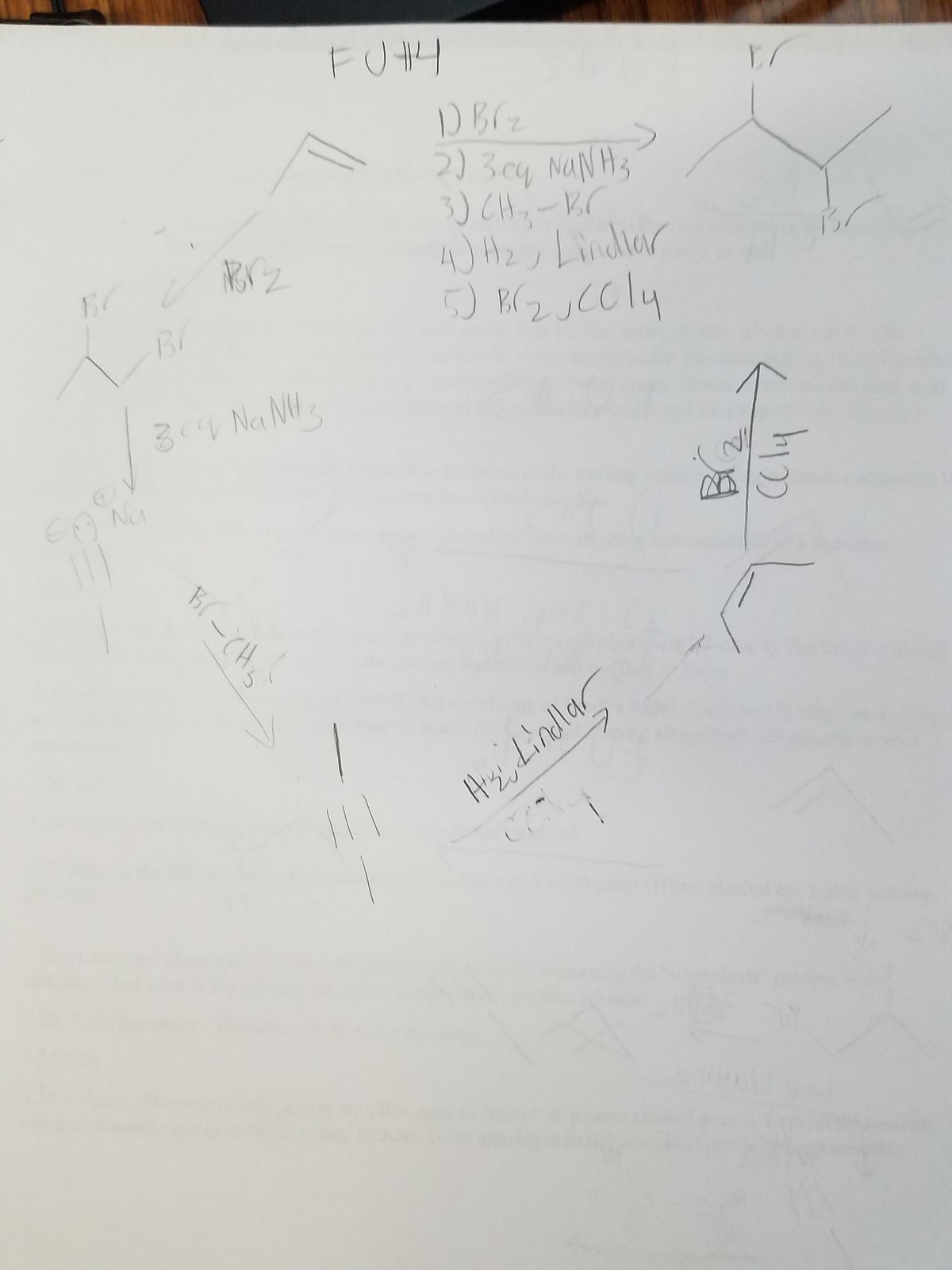The image depicts a handwritten set of notes detailing a chemical reaction sequence, scribbled on a piece of white scratch paper. Evident typing can be seen faintly from the other side of the paper, while a subtle background strip runs across the top, hinting at incomplete print or shadowing.

At the top center, penciled in large letters, is "FU number 4," below which a numbered list from 1 to 5 details various chemical reagents and conditions:
1. BR2
2. 3CQNANH3
3. CH3 - BR
4. H2 with LINDAR (Lindar Catalyst)
5. BR2 with CCL4

To the right of item 1 ("BR2") is an outlined partial molecular structure. It begins with a hexagonal ring, where one vertex is extended upwards into a spike labeled "FR" and another labeled "BR" descends diagonally to the lower right.

On the left, adjacent to the list, a sequence of reaction steps is sketched. It starts with:
- A double-line arrow pointing upwards to "BR2" followed by a downward arrow aligned with lines reaching up and down, terminating in "BR".
- Continuing from "BR2," the pathway uses consecutive steps with reagents like NANH3, breaking down into NA. 
- An arrow from NANH3 leads to the "BR - CH3" step, branching into multiple lines.
- Farther to the right, the reactions involve "H2 LINDAR" transitioning through angular lines signifying molecular transformations.
- Finally, an arrow leads up and over to the notation of "BR2 with CCL4" indicating the last step in the process.

Overall, this intricate schematic outlines a detailed chemical reaction pathway associated with "FU number 4," meticulously reflected in schematics and notations critical for understanding the multi-step synthesis or reaction process.